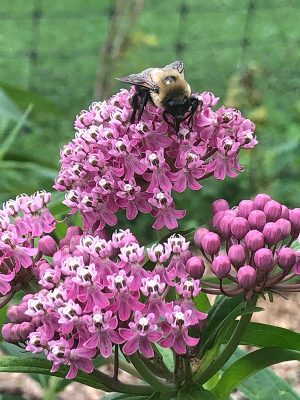The photograph captures a captivating purple flower in full bloom. The multi-headed flower forms a rounded cluster composed of numerous small blossoms, each showcasing a pinky-mauve hue. Some of the blossoms are fully open, revealing delicate white centers that are raised and likely teeming with pollen. At the pinnacle of the flower cluster, a sizable bee is perched, busily collecting nectar from the tallest bloom. To the lower right of the image, an unopened section of the flower is visible, hinting at the intricate structure of many individual stems and blossoms yet to bloom. The image beautifully encapsulates the delicate interplay of color, texture, and life in the floral world.